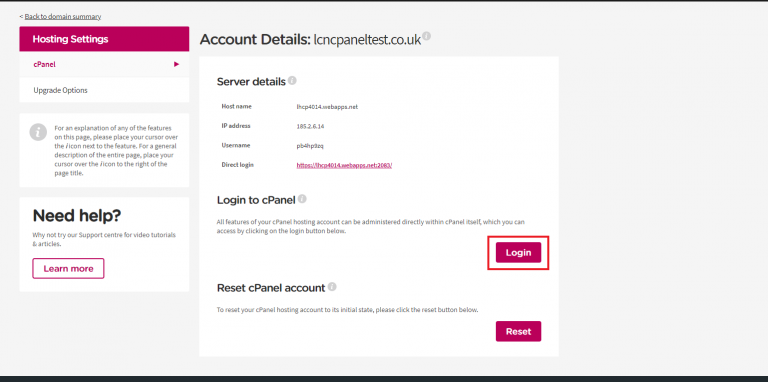This image depicts a screenshot of a computer screen displaying account details for a hosting service. The background is gray, and various sections are highlighted by white rectangles and squares. In the upper left corner, there's a link labeled "Back to Domain Summary." Directly below it, a pink rectangle reading "Hosting Settings" is prominently displayed. 

Descending further down the left side, a "cPanel" button is followed by an "Upgrade Options" button. Central to the image, at the top of the primary section, is the heading "Account Details" with the domain "lcncpaneltest.co.uk" specified underneath. 

Below this, a white square titled "Server Details" lists information such as the hostname, IP address, username, and direct login credentials. Another section titled "Login to cPanel" explains that all features of the cPanel hosting account can be managed directly within cPanel, accessible by a login button below. This login button, pink and outlined in red, is situated immediately after the explanatory text.

Beneath the login button, instructions for resetting the cPanel account are provided, accompanied by a pink "Reset" button. To the left of these options, there's a "Need Help?" section with a clickable "Learn More" button to assist users in navigating their hosting settings.